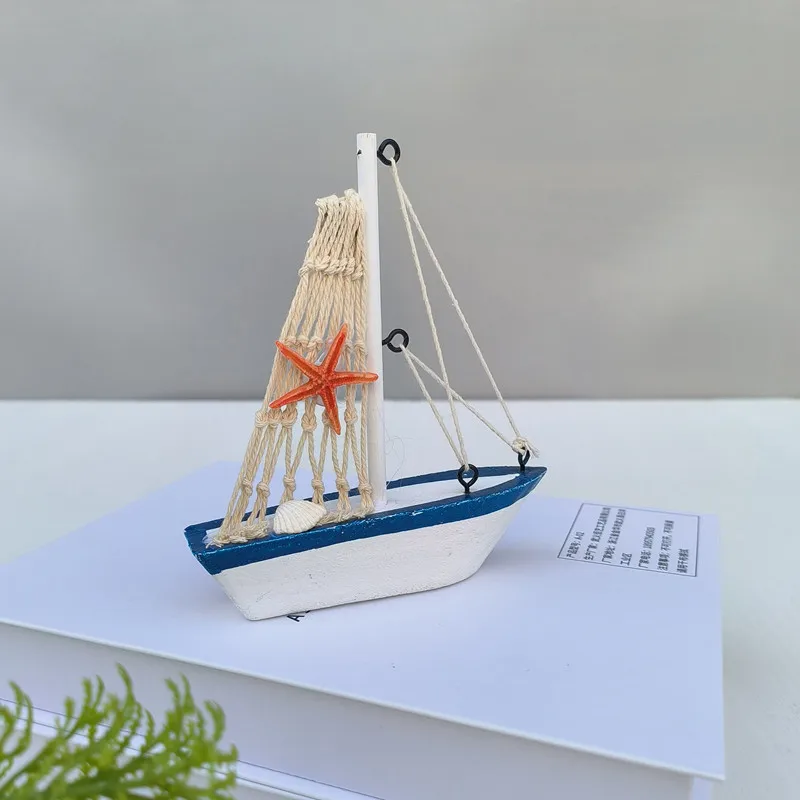The photograph depicts a scene with a gray wall as the background and a small tabletop or surface in the foreground. In the lower left corner, partially obscured and cropped out of full view, there is a plant with green leaves adding a touch of nature to the image. Dominating most of the table's surface is a detailed model of a miniature sailboat. The boat itself is white with a blue trim along the edges, evoking the appearance of a handcrafted kit assembled with care. Central to the boat is a white mast with tan strings representing the rigging and sail lines that crisscross the structure. Adorning the sail is a small, bright reddish-orange starfish, and at the base of the mast lies a delicate white seashell, adding a whimsical and decorative touch. The boat rests atop what appears to be an envelope or a booklet, though the text on it is small, facing away from the camera, and indecipherable. The overall composition combines elements of craftsmanship with hints of nautical and natural themes, set against a minimalist backdrop.